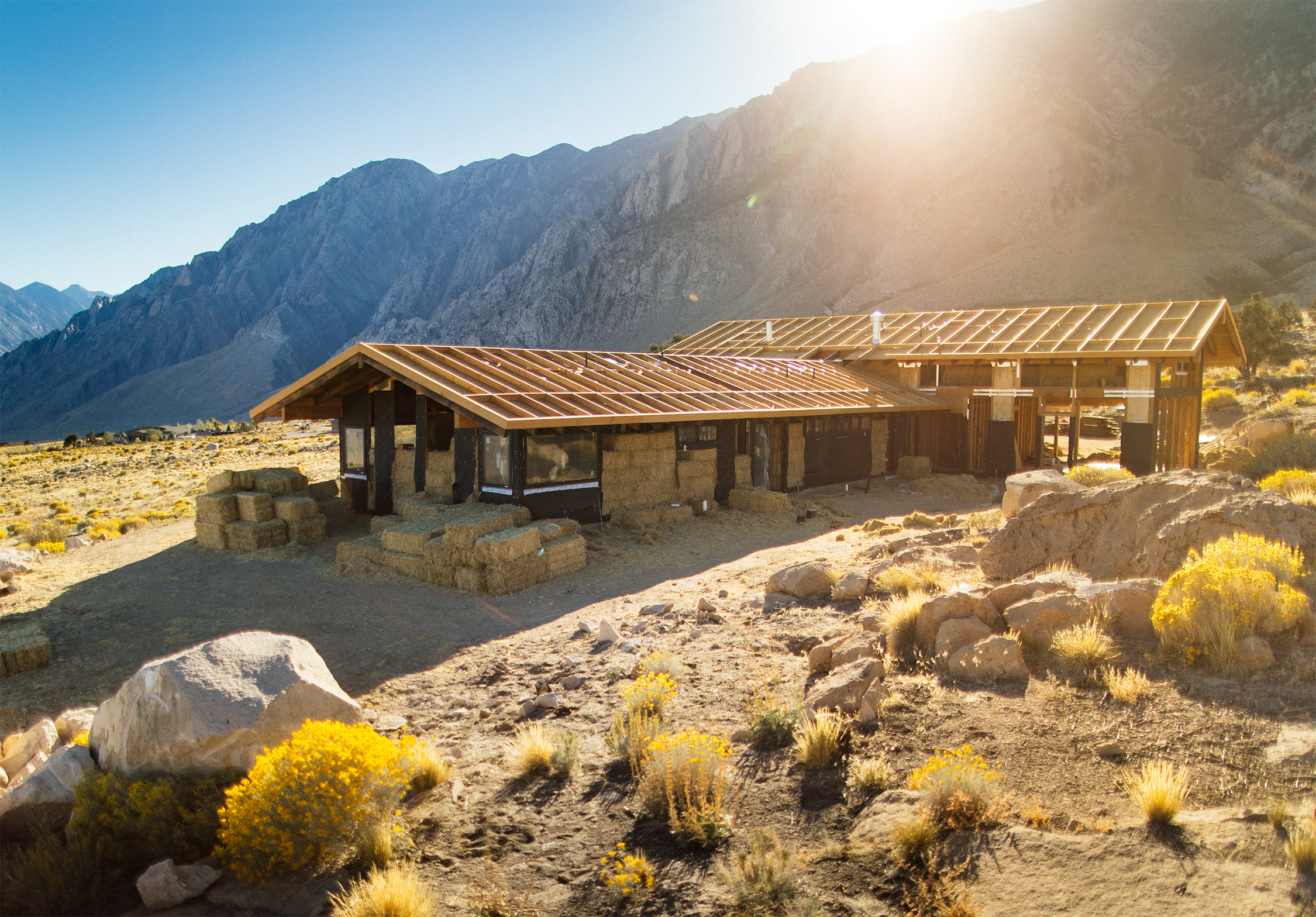In the image, there appears to be a barn under construction or renovation, situated in a rugged and dry landscape. The barn, shaped roughly like a "T," features framed but unfinished walls and an exposed wooden beam roof. The barn is filled with hay bales, with more bales stacked outside one end. Surrounding the barn is a stark, barren terrain of rock, sand, and sparse vegetation, including occasional yellow-flowered shrubs and tumbleweeds. The ground immediately around the barn is cleared, revealing exposed dry dirt. In the background, a large mountain ridge looms, with the sun beginning to rise above it, casting early light onto the scene.